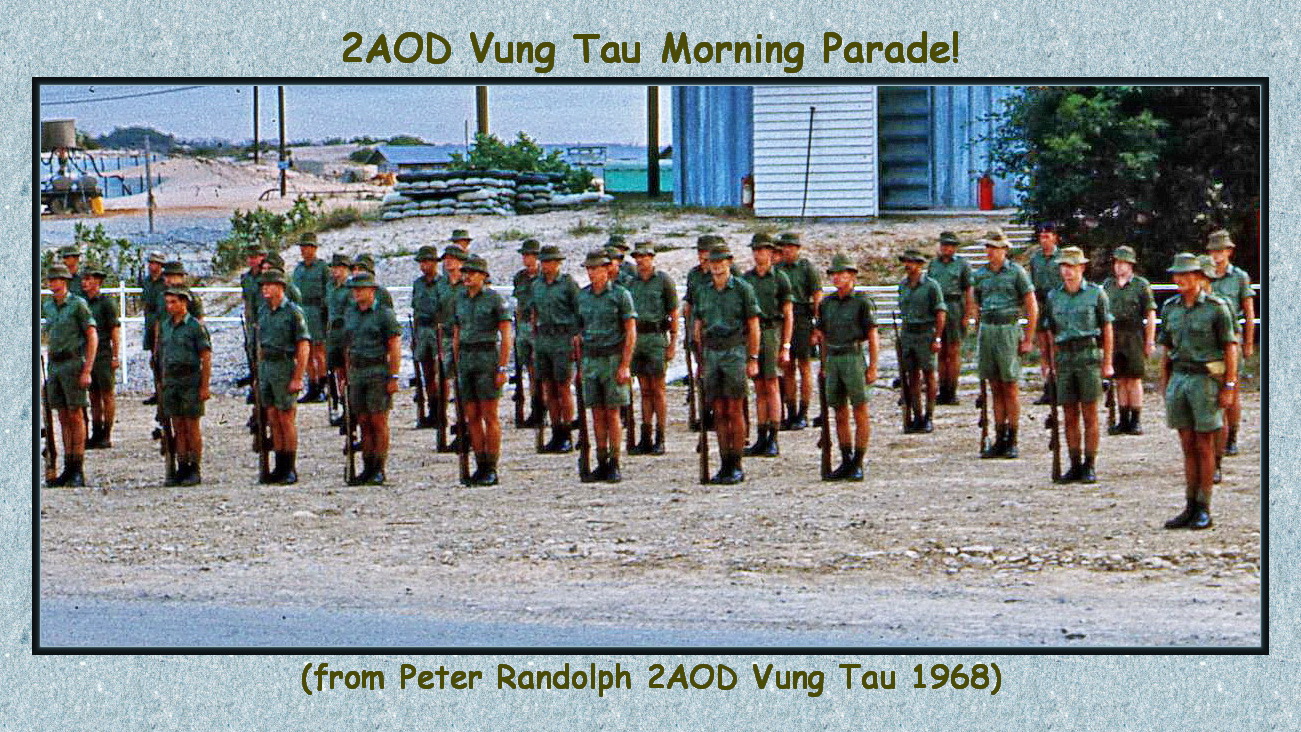This color photograph, set within a light blue border, features a morning parade of soldiers from AOD Vung Tau, 1968. The headline at the top reads "To AOD Vung Tau Morning Parade!" and the bottom caption states "From Peter Randolph to AOD Vung Tau 1968" both in dark green type. The image, in landscape orientation, showcases a platoon of soldiers standing in several rows on a dry, dirt-covered ground. Clad in dark green short-sleeved shirts, shorts, and matching hats—although a few wear tan hats—the soldiers stand at attention with rifles held upright at their right sides and black shoes on their feet. In the backdrop, a blue building and several telephone poles stretch across the middle, with trees on the right side and a hint of water to the left. The overall scene is captured in a style that merges photographic realism with elements of graphic design, providing a vivid historical snapshot of the disciplined military formation.